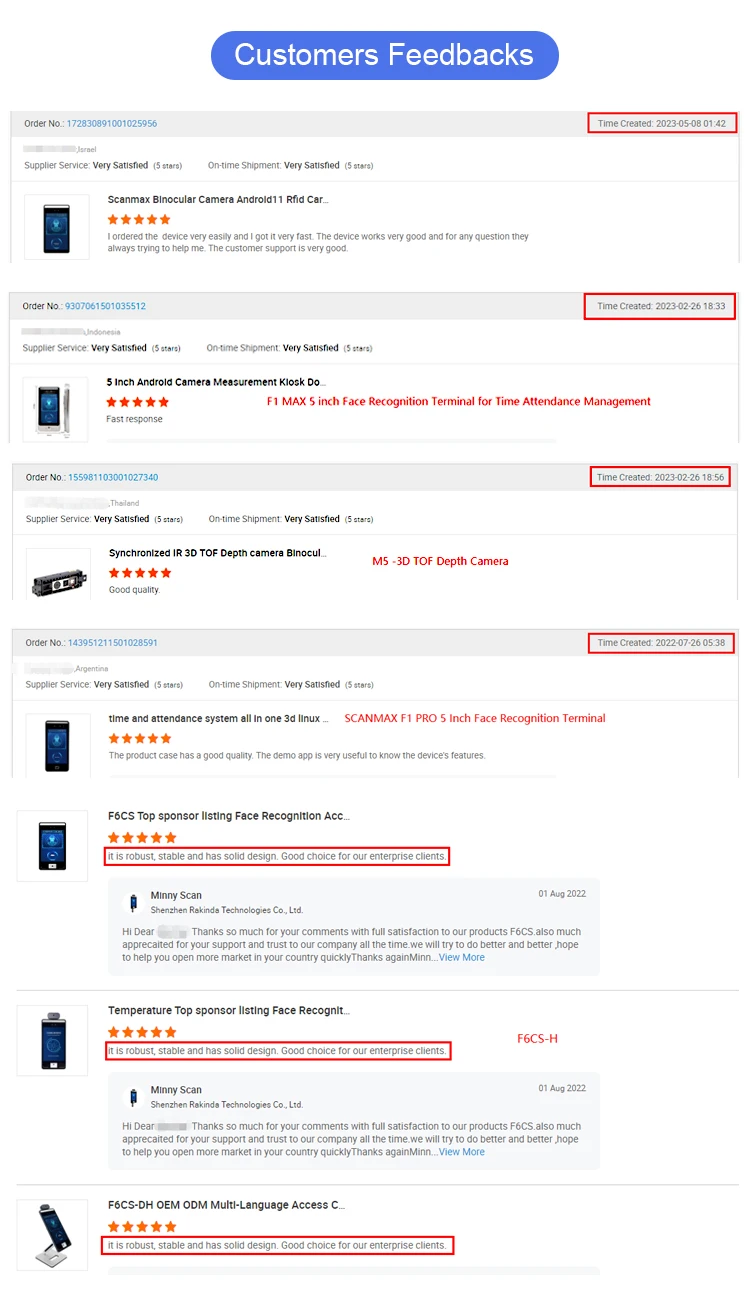The image captures a bright web page with a predominantly white background. At the very top, there is a horizontal blue cylindrical banner featuring a baby blue box in the center, adorned with the words "Customer Feedbacks" in white font. Below this banner, a section dedicated to user reviews is displayed. This section showcases various devices, likely cell phones and tablets, though the details are somewhat unclear due to the small size of the images.

On the left-hand side of the section, small images of the devices are arranged, possibly categorizing the feedback according to different models. On the far right-hand corner, thin red rectangular boxes are visible, each containing gray font text that appears to denote the purchase date and price, though the specifics are difficult to discern. The entire layout seems to provide a list of customer reviews with corresponding device images and purchase details.